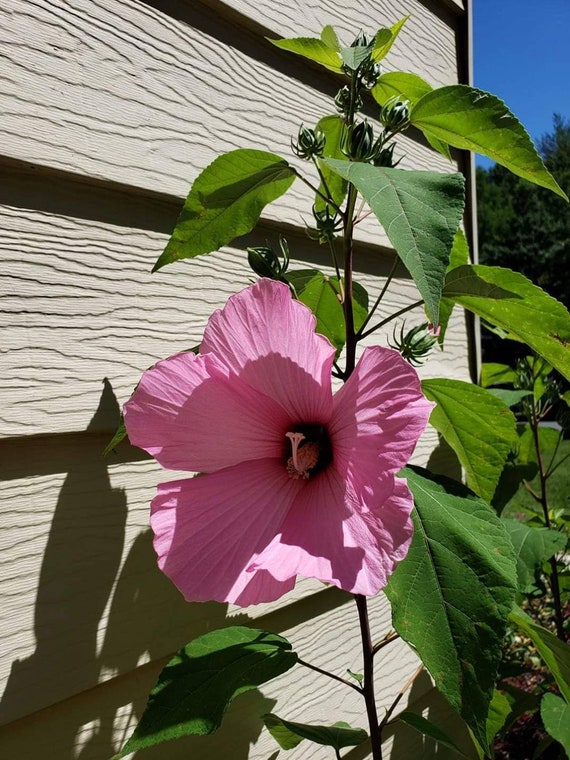The image depicts a beautiful, large pink hibiscus flower in full bloom, positioned in the center against the backdrop of gray siding from a house. The flower is the centerpiece, surrounded by an abundance of green leaves and several buds poised to blossom. The bright, sunny day casts distinct shadows of the hibiscus and its foliage onto the house siding, enhancing the vividness of the scene. Above the flower, a strikingly blue sky and leafy green trees can be seen in the upper right corner, suggesting a suburban setting with a well-kept lawn in the background. The sunlight streams from behind the flower, enriching its vibrant pink hue and highlighting the intricate details of the flower's central stem.